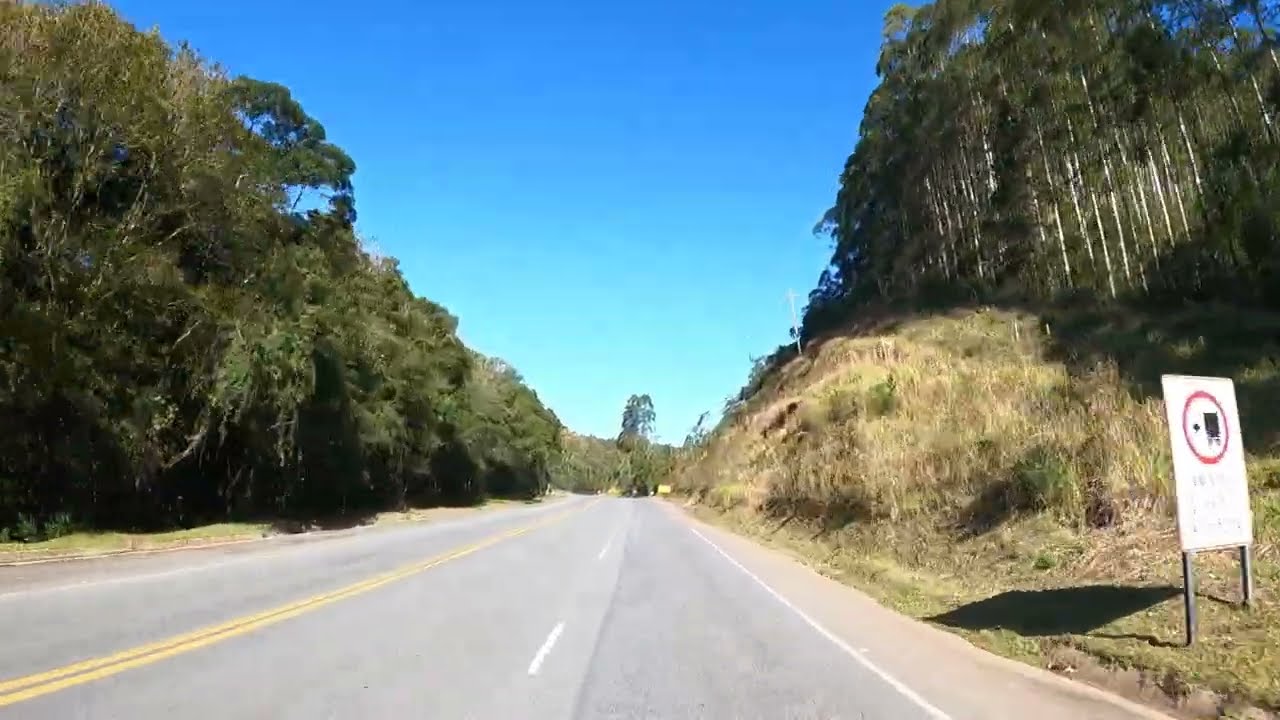This photograph captures a four-lane road on a bright, clear day, with the sky transitioning from a turquoise hue near the horizon to a deeper blue higher up. The road is distinctly divided by two solid yellow stripes down the center and white dashed lines between the lanes. On the right side, a white sign with a red circle and an indistinct black object stands near the base of a hill, which is covered in grass and weeds, and crowned by tall trees with white trunks. The left side of the road is lined by slightly shorter, thick-leaved trees. The road stretches into the distance, where more trees blend into the horizon, including one particularly tall tree that rises prominently above the others. Notably, there are no vehicles visible on the road.